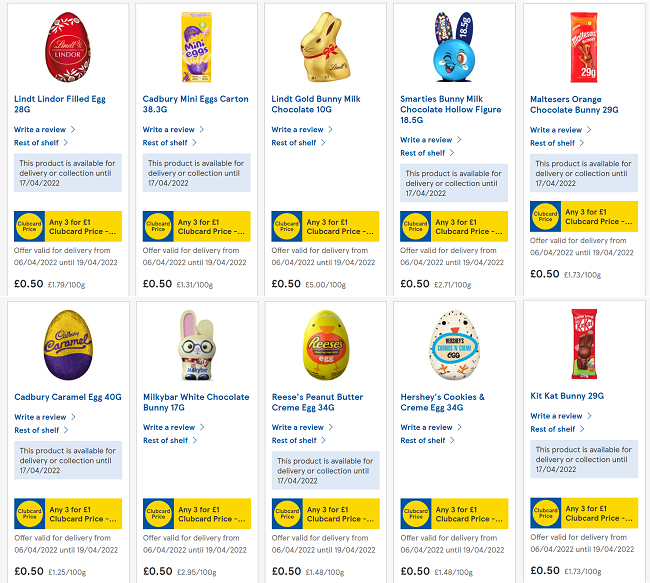Screenshot of a website displaying a search result page for "chocolate eggs." The page is organized into two rows, each containing five products. Each product listing includes an image of the chocolate egg or Easter bunny, the title of the item, and a "Write a review" link in blue text with a small arrow next to it. Beneath this, there is another blue text link that says "Rest of shelf," also accompanied by a small arrow.

For seven out of the ten products, there is a gray box stating, "This product is available for delivery or collection until 17-04-2022." Below this box, each product has a yellow button with a blue-outlined circle on one end, displaying the message, "Any 3-for-1 Clubcard Price." The offer for the Clubcard price is valid from 6-04-2022 until 19-04-2022.

Each product is priced at 50 cents, with the unit price listed next to it. All the products appear to be variations of Easter bunnies or Easter eggs.